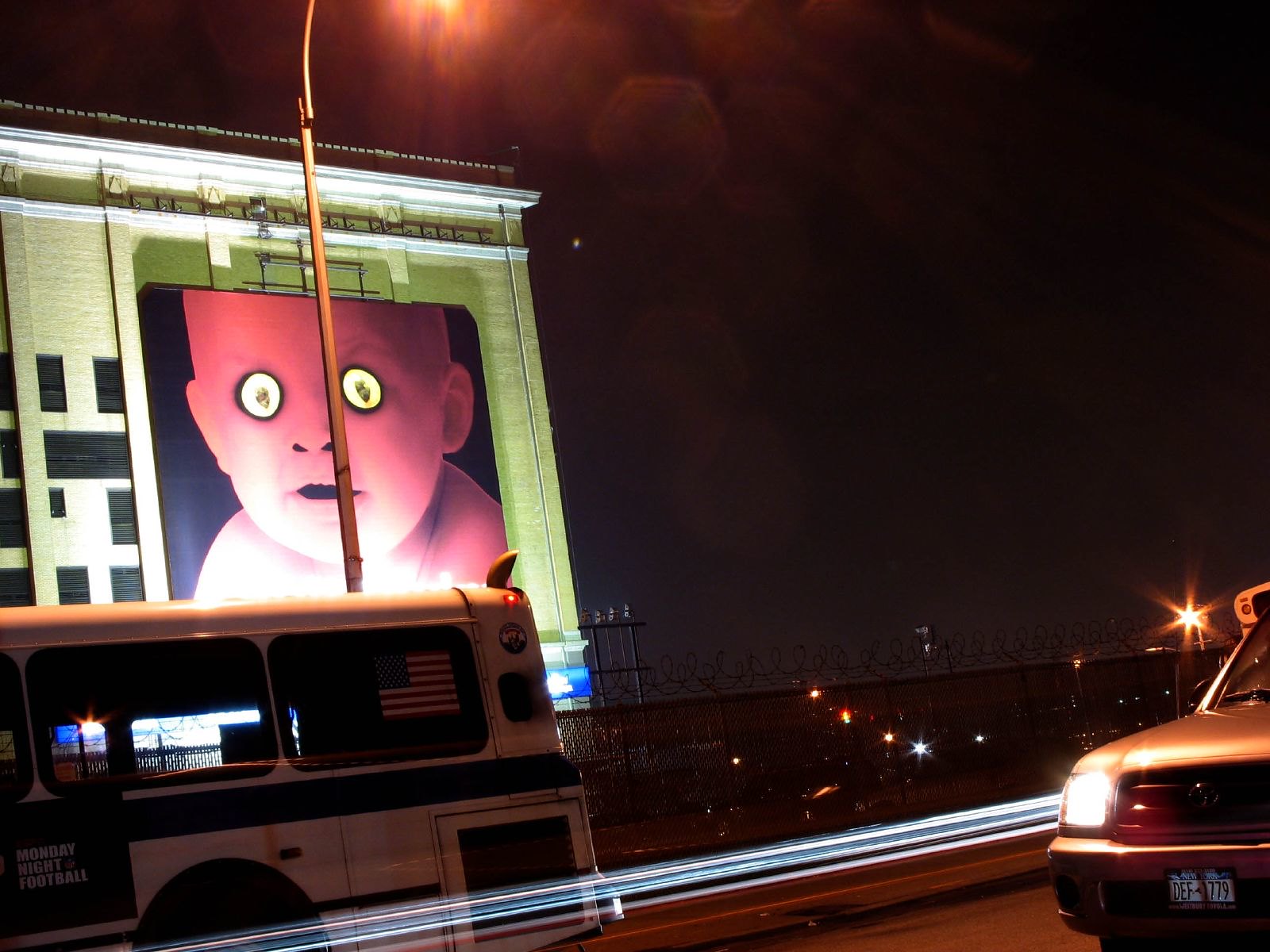A nighttime photograph captures a dimly lit urban street scene. On the bottom right, the front left side of an SUV is visible, its headlights illuminated and license plate displayed. The bottom left corner of the frame includes the rear end of a white bus, with its final two windows and the wheel well, though the wheel itself is not visible. A streak of light cuts through the middle of the scene, a motion blur from another passing vehicle or light source.

A spiked, "do not cross" security fence stretches along the road, its menacing barbed wire glistening under the scant light. Behind this fence, a tall building looms with a large, unsettling advertisement of a baby's face. The baby's eyes appear like eerie cucumbers, and its nostrils and mouth are dark voids against a black background, giving the poster an unnerving, painted-on appearance.

Streetlights illuminate portions of the street and the tops of the two vehicles. In the background, to the right, city lights from lower buildings twinkle behind the fence, though only hints of the cityscape are visible due to the low angle of the shot. The top center of the image is adorned with a bokeh effect caused by the streetlights glowing softly against the night sky.